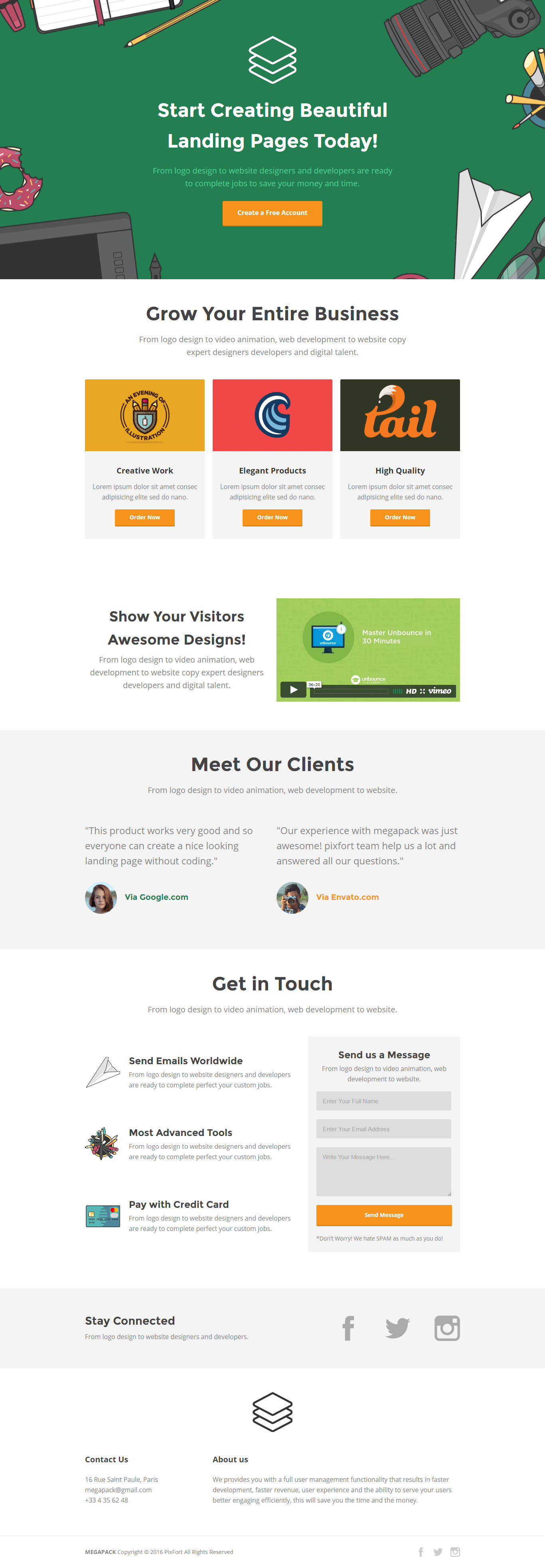**Detailed Caption for Web Page Screenshot:**

The screenshot captures a comprehensive web page designed to promote Megapack's services. 

**Header Section:**
- The topmost part features a vibrant green background with scattered clip art icons. The bold headline reads, "Start creating beautiful landing pages today," followed by a subtext: "From logo design to website designers and developers, ready to complete jobs to save your money and time." A prominent button below invites users to “Create a Free Account.”

**Main Section:**
- Beneath the header, a white background section states, "Grow your entire business from logo designs to video animation, web development to website copy, expert designers, developers, and digital talent."

**Feature Boxes:**
- Center-aligned are three feature boxes:
  - **Left Box:** Orange background featuring an event titled “An Evening of Illustration” with a clip art pocket containing pencils. Below it reads "Creative Work" followed by some placeholder Latin text and an "Order Now" button.
  - **Center Box:** Red background with a wave icon. It is labeled "Elegant Products" with placeholder text and an "Order Now" button beneath.
  - **Right Box:** Black background with a logo saying "TAIL" in artistic orange script, the 'T' stylized with a fox tail. It is labeled "High Quality" with placeholder text and an "Order Now" button.

**Video Section:**
- Below the feature boxes, another section encourages showcasing designs: "Show your visitors awesome designs from logo design to video animation, web development to website copy, expert designers, developers, and digital talent." To the right, there is an embedded Vimeo video titled "Master Unbounce in 30 Minutes."

**Client Testimonials:**
- Following the video section, a gray background area titled "Meet Our Clients" features testimonials:
  - The left testimonial reads, "This product works very good, enabling everyone to create a nice-looking landing page without coding," accompanied by a generic woman’s picture labeled via Google.com.
  - The right testimonial states, "Our experience with Megapack was just awesome, PIX14 helped us a lot and answered all our questions," accompanied by a man’s picture with a camera, labeled via Envato.com.

**Contact Section:**
- On a white background, the "Get in Touch" section includes:
  - Three contact options with clip art images for sending emails, using advanced tools, and paying with a credit card, each accompanied by text repeating readiness to perfect custom jobs.
  - To the right, a text box for sending messages is provided, requesting full name, email address, and message, with an assurance against spam.

**Social Media and Contact Info:**
- Below, a gray section titled "Stay Connected" features Facebook, Twitter, and Instagram logos.
- Following this, a white background section provides contact info: "Contact us at 16 Rue St. Paul Paris, Megapack at gmail.com," with a phone number and an "About Us" section detailing user management functionalities.

**Footer:**
- The bottom of the page shows Megapack's copyright information: "© 2016 Pixfort All Rights Reserved," along with Facebook, Twitter, and Instagram symbols.

This detailed caption encapsulates the layout, design, and key elements of the captured web page, providing a clear and comprehensive description.